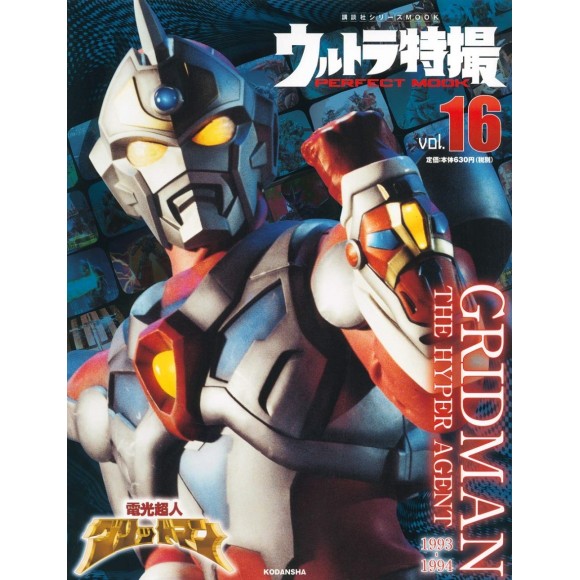The image is a cover of a Japanese comic book titled "Gridman the Hyper Agent". It prominently features a lifelike humanoid robot that resembles a character from Power Rangers, with its left hand curled into a fist. The robot has humanoid features with glowing yellow eyes, a blue pointy appendage sticking out of its head, and a red diamond-like emblem in its chest. There is detailed text on the cover, with Japanese characters at the top and the bottom, and English text running vertically along the right side that reads, "Gridman the Hyper Agent 1993 to 1994." It also notes "Perfect Mook Volume 16". The text "B-O-L" in white and "16" in red is visible at the top. The cover is adorned with a mix of bright red and yellow accent colors and multiple gadgets integrated into the robot's suit, hinting at its combat capabilities.